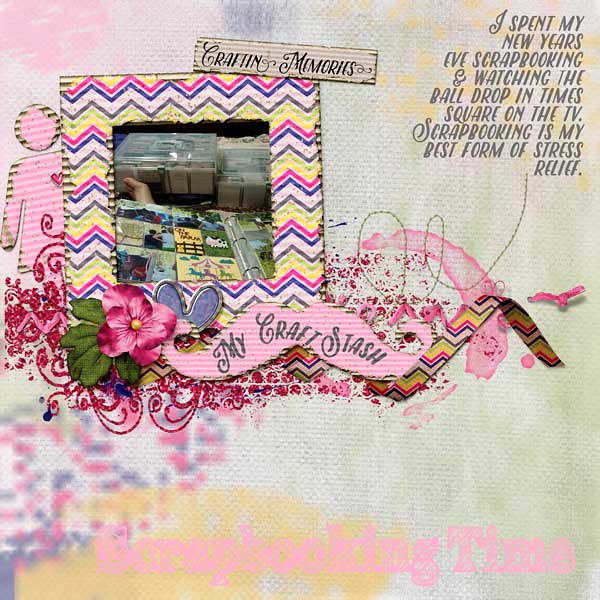This vertically oriented image features a creatively composed scrapbook page set against a predominantly pale green background. The centerpiece of the composition is an assortment of artistic elements, including florals and abstract designs, characterized by a blend of vibrant pink, blue, white, brown, green, and yellow hues. 

At the top of the image, the phrase "Crafting Memories" is prominently displayed. Below it, there is a square filled with squiggly lines in pink, blue, white, and brown, framed by additional colorful accents in green and yellow. Nestled to the left of this square is a cluster of green, red, and purple flowers.

Further down, the phrase "My Craft Stash" is featured prominently, possibly on a pink mustache shape, while the lower section is adorned with elegant, faded dots of blue, yellow, pink, and purple. To the left of the floral arrangement, there's a delicate outline image of a woman in a dress, rendered in pink.

In the upper right corner of the image, gray text reads: "I spent my New Year's Eve scrapbooking and watching the ball drop in Times Square on the TV. Scrapbooking is my best form of stress relief." This text is an indication of the creator's passion for scrapbooking and the therapeutic value it holds for them. The text "Scrapbooking time" is also visible towards the bottom, emphasizing the theme of the artwork and the enjoyment derived from this creative hobby.